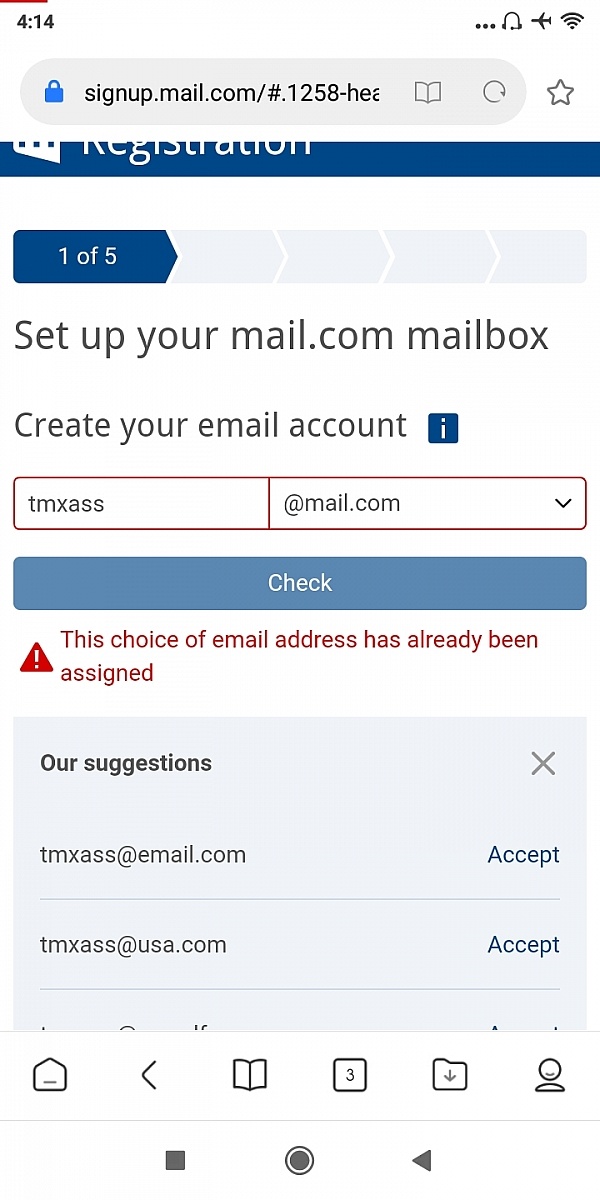The image is a screenshot with a white background. In the top-left corner, the time is displayed as 4:14. On the top-right corner, there is a black outline featuring a notification bell, an airplane mode icon, and a Wi-Fi icon. Below this, there is a web address bar in a light gray rectangle with rounded corners, containing a blue padlock icon indicating a secure website. The URL reads "signup.mail.com/#1258-HER," though some parts of the text are not legible.

Further down, partially visible against a blue background with white letters, is the word "registration." To the left, there's a small blue rectangle with a pointed end on the right that reads "invite 105."

In the central portion of the image, against a white background, the text in black font reads "set up your mail.com mailbox. Create your email account." Below this, there are two text input boxes side by side. The left box has "TMXASS" entered, and the right box is fixed with "@mail.com." 

Beneath these input fields is a lighter blue rectangle with "check" written in white in its center. Below this button, there's a red warning message featuring a red triangle with a white exclamation mark, stating: "The choice of email address has already been assigned."

Finally, at the bottom of the screenshot, in black text, it reads, "our suggestions: TMXASS@mail.com and TMXASS@USA.com."